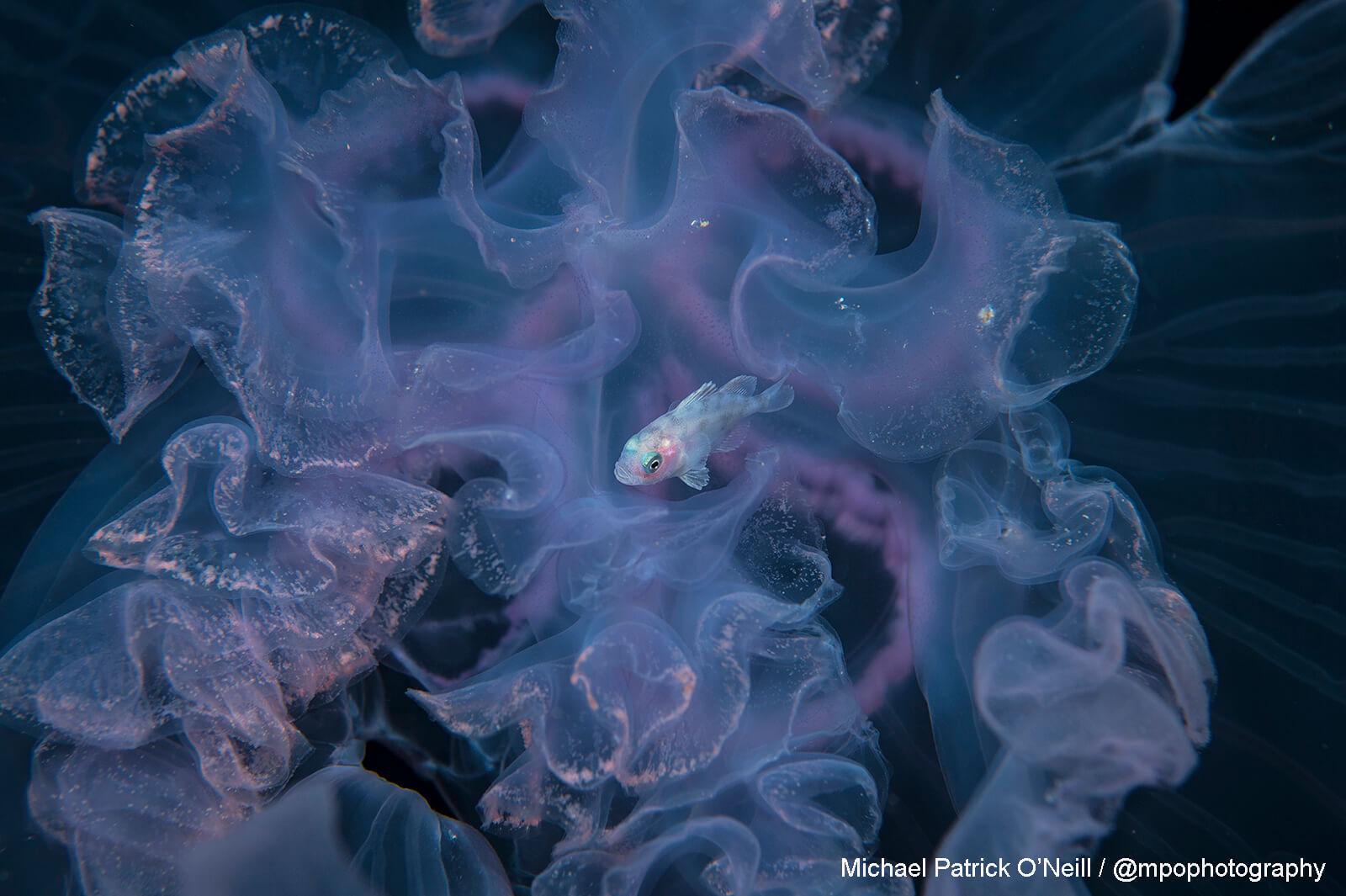This underwater photograph by Michael Patrick O'Neill, captured in deep, dark blue waters almost appearing black, features a small, translucent fish surrounded by what seems to be a large jellyfish or a group of jellyfish. The fish, about the size of a goldfish, has delicate features with a predominantly white body that is tinged with green behind its eye and pinkish hues near its gills. Its eye is black, encircled by blue, and it has light gray, tiger-stripe-like patterns down its back. The jellyfish-like creature enveloping the fish has a flowing, wavy texture with predominantly purplish-blue tones accented by strands of fluffy pink. Its translucent, layered edges create a mesmerizing, almost ethereal appearance. The photograph exudes a cool, serene aura with its detailed textures and colors. In the lower right corner, the image is signed with "Michael Patrick O'Neill @ MPOP Photography" in white text, highlighting the artist's name and handle.